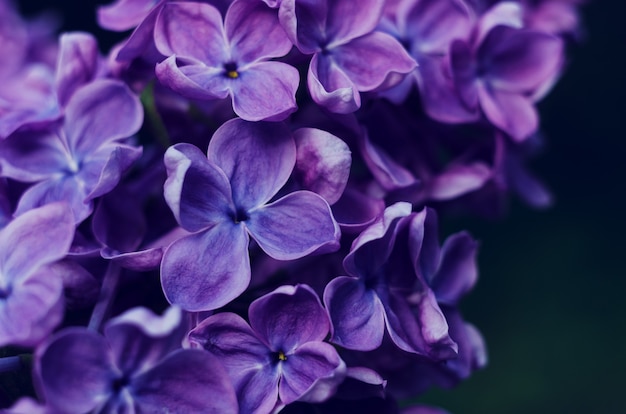This is a detailed, close-up nature photograph of small purple flowers, possibly African violets or hydrangeas, taken outdoors. The flowers, with their striking variety of hues and intricate petal patterns, are the focal point of the image. Each bloom typically has four teardrop-shaped petals that curl inward towards the center, giving them a delicate, bowl-like appearance. The petals display a spectrum of purples, from light lavender to deep magenta, and many show subtle striations and color variations, ranging from purpley blue to a more solid purple. The centers of the flowers either feature a contrasting yellow spot or a dark blue spot. White areas are also visible among the flowers, potentially indicating a transitional phase in their color development. The background is dark, possibly black or blue, creating a sharp contrast with the vibrant flowers. It is mostly out of focus, but a hint of green is visible in the upper right corner, suggesting the presence of greenery. The sharp clarity of the blooms in the foreground gradually blurs towards the back and sides of the image, emphasizing the depth and richness of the floral display.